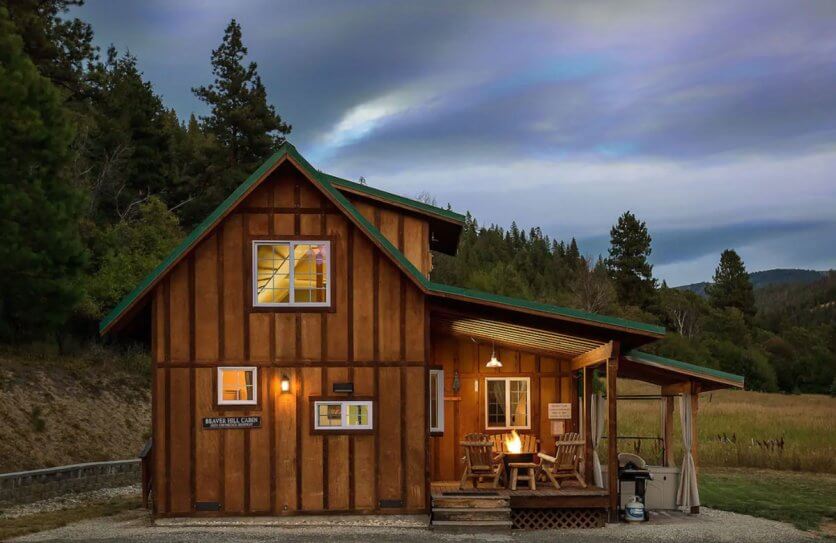The photograph captures a charming, cozy wooden cabin with a green roof, situated amidst a vibrant forest. Taken during sunset, the cabin emanates a warm, inviting glow from its well-lit interior. The structure features dark brown wooden slats and is adorned with beige curtains. A wooden deck at the front displays several chairs and a grill with propane underneath, emphasizing a homely atmosphere. A sign on the left side reads "BEAVER HELD CABIN" in white capital letters against a brown background. The porch showcases a hanging light and a small fireplace, adding to the rustic charm. Surrounding the cabin is a mix of green grass and tall, dark forest green evergreen trees, enhancing the picturesque woodland setting.